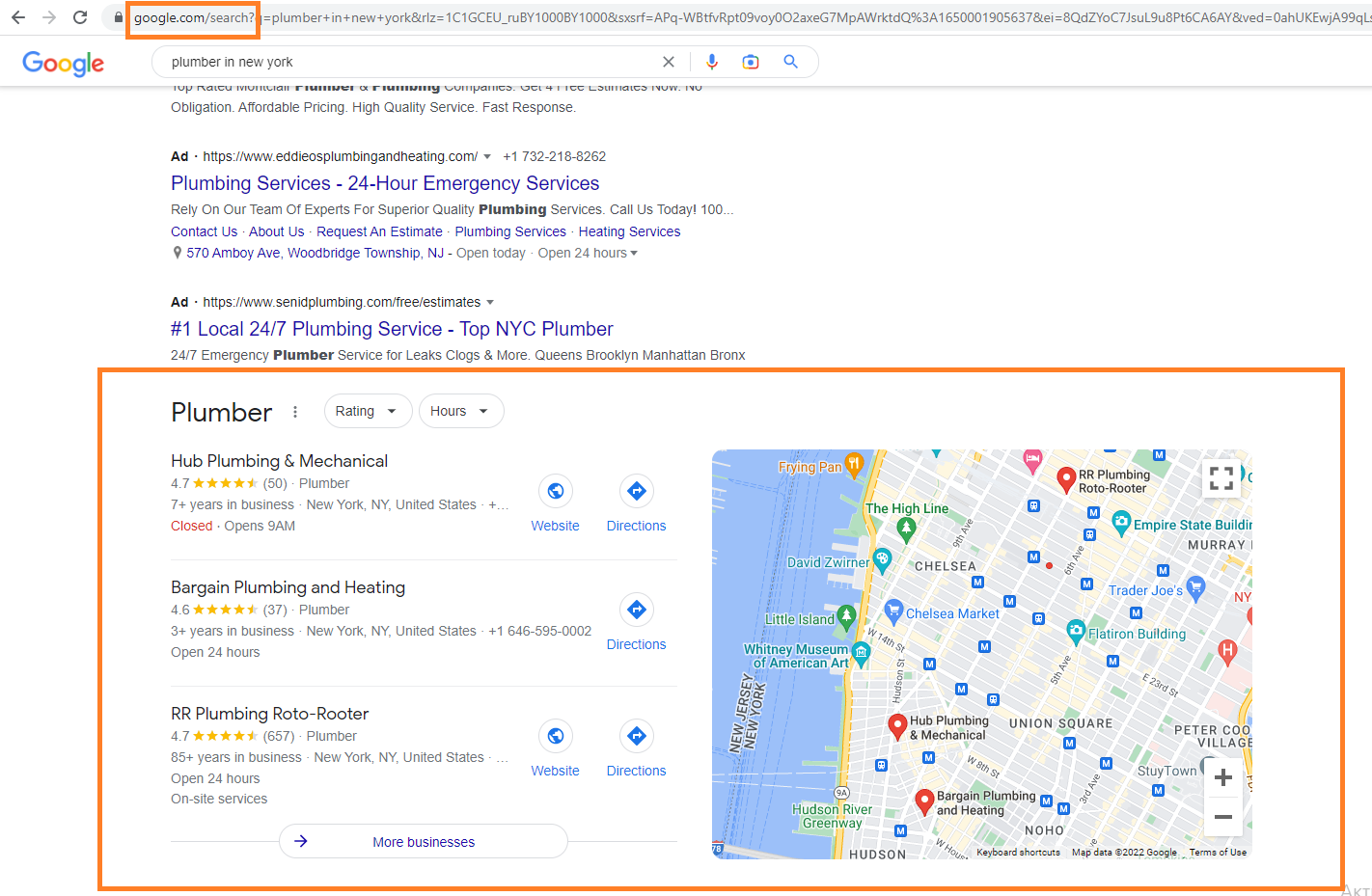The image depicts a Google search results page shown in a left-to-right horizontal orientation. The background is predominantly white, reflecting the computer screen's display. At the top of the screen, navigation buttons are visible, including a clickable "Back" button, a grayed-out "Forward" button, and a "Refresh" button, alongside the search bar. The URL in the search bar, "google.com/search", is highlighted with an orange box. 

To the left of the search bar, Google's traditional colorful logo is prominently displayed. Below the URL bar, the search field contains the query "Plumber in New York", with accompanying icons for voice search (microphone), image search (camera), and the search action button (magnifying glass). 

The search results include several advertisements, each featuring essential information such as the web address, title, phone number, business details, and operating hours. A section titled "Plumber" presents different options encased in an orange rectangular box. This section includes business names such as Hub Plumbing and Mechanical (rated 4.7 stars), Bargain Plumbing and Heating (rated 4.6 stars), and RR Plumbing Roto-Rooter (rated 4.7 stars). Additional details provided are the number of reviews, years in service, and specific locations, with options to visit the website or get directions.

To the right of the search results is a map displaying the geographical locations of the listed plumbing services in New York. The map provides a visual reference for the user to pinpoint the businesses' physical locations.